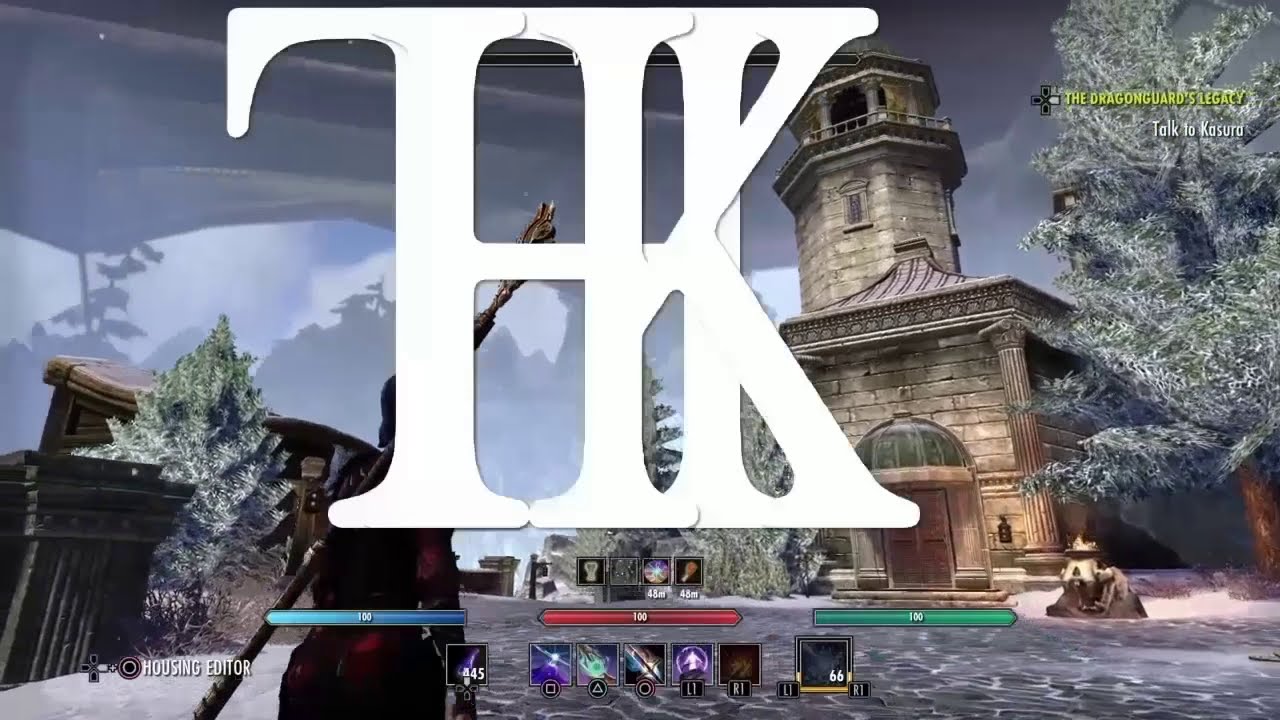In this detailed screen capture from a fantasy role-playing game, set within a context that evokes medieval or Asian architectural themes, we see a character clad in red armor with an ambiguous, staff-like weapon strapped across their back. The character is positioned slightly to the middle left, partially obscured by large, overlapping white letters—likely forming the acronym "THK" or "TFK"—which dominate the frame. The scene depicts a tranquil yet atmospheric environment, complete with snow-covered pine trees and an ornate stone building or temple prominently in the background. The gameplay interface includes three meters at the bottom, colored blue, red, and green, indicative of different resources or powers available to the player, alongside icons for various spells or actions. In the top right corner, quest guidance text reads "The Dragon Guard's Legacy. Talk to Kasura," tying the visual elements to a narrative direction within the game. This image captures the intricate design and immersive elements typical of a high-fantasy RPG experience, potentially by a well-known developer like Bethesda, with visual cues suggesting it is a console version.